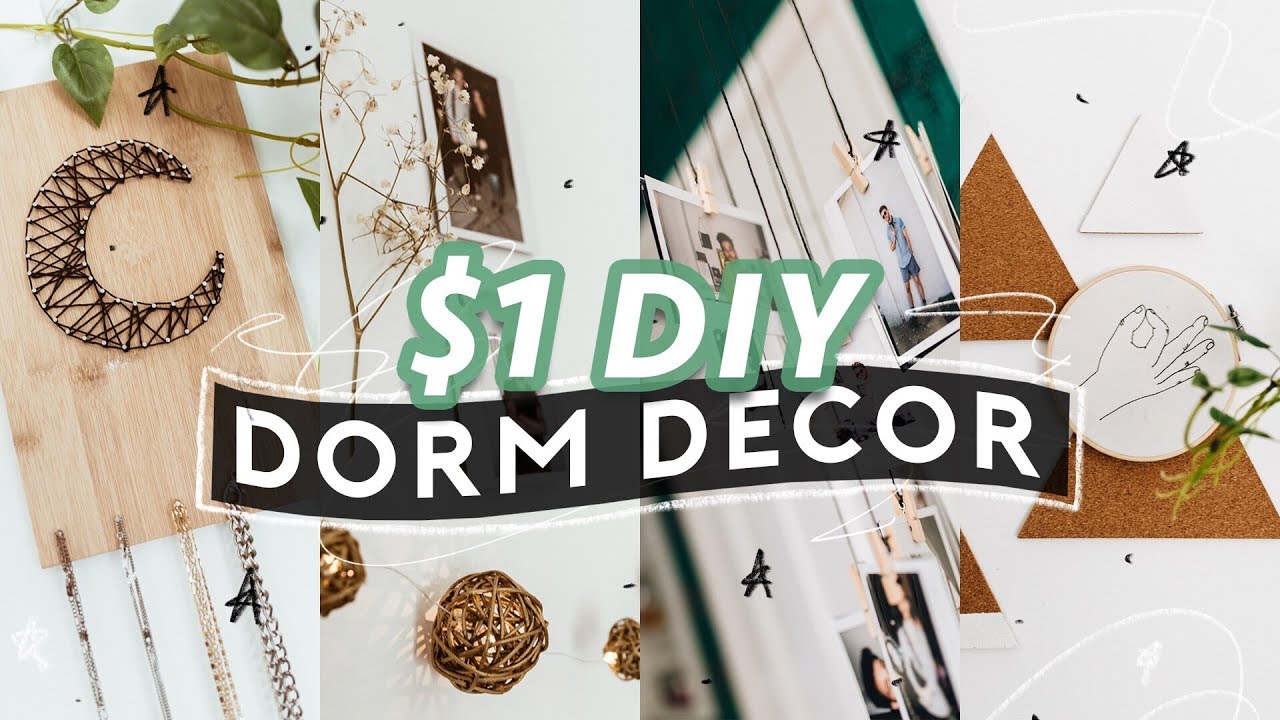The image is a vibrant and inviting advertisement for DIY dorm decorations. Centrally displayed on a predominantly white background, bold, multicolored text reads "$1 DIY" in a striking green-bordered white font, and "dorm decor" in a stylish black-bordered white font. Surrounding the text are an array of charming dorm decor items. 

In the top left corner, a vine with green leaves adds a touch of natural elegance. Below it, a light-colored wooden board features a metal decoration shaped like a crescent, with various necklaces elegantly draped from hooks resembling an artistic jewelry display. 

To the right, a creative display shows framed photographs affixed to a black string by clothespins, lending a personal touch. A moon-shaped thread trinket is adorned with more necklaces, adding to the celestial charm. Complementing these elements are faint, whimsical white doodles and scribbles that enhance the overall playful aesthetic.

The image also features additional enchanting items, such as a dried flower book press, bronze wall ornaments, and a photograph, rounding out the diverse decor selection. The main colors showcased include white, turquoise, navy blue, and natural tones, creating a coherent and appealing color scheme ideal for dorm room inspiration.